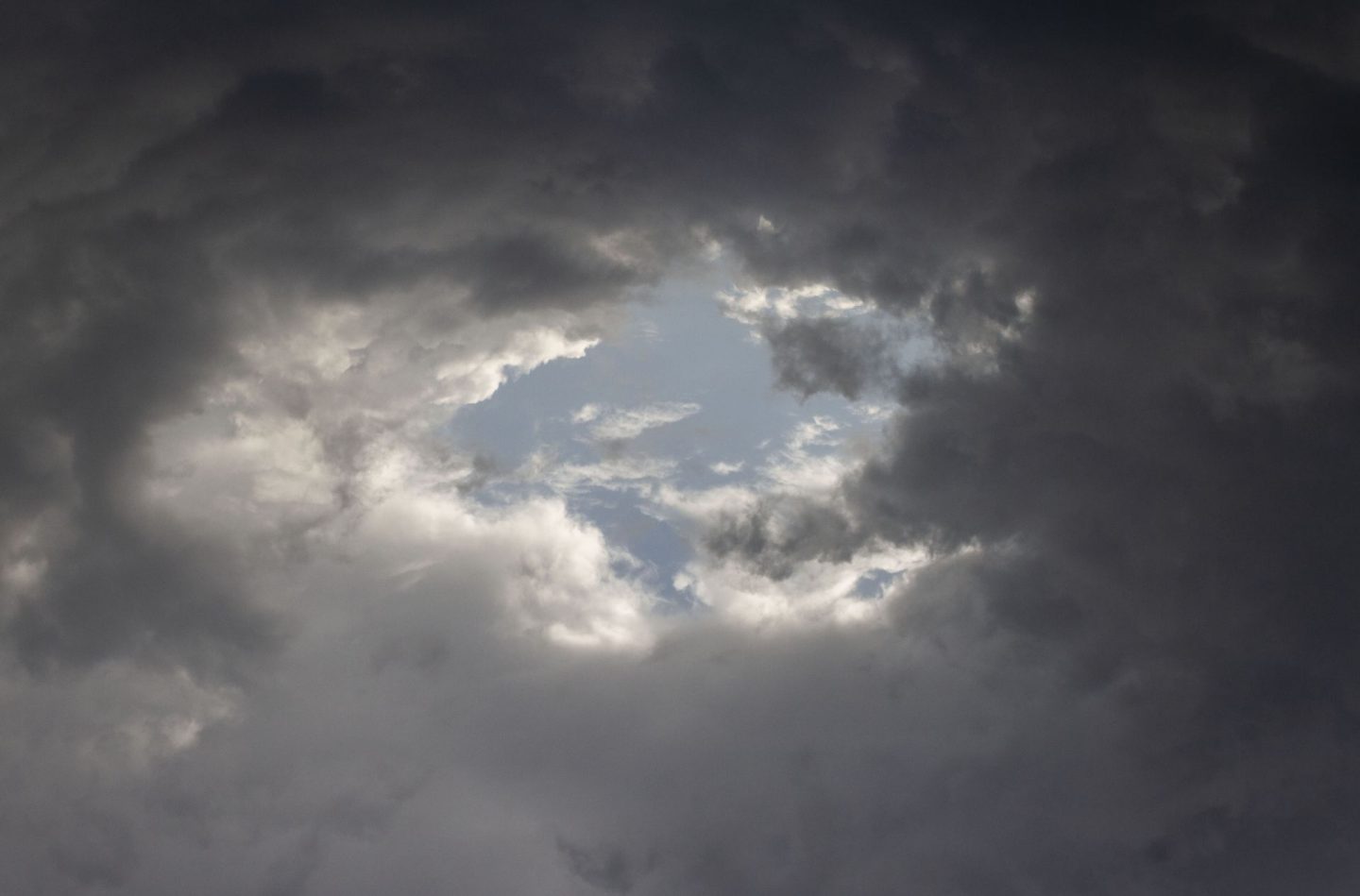The image captures a dramatic and ominous sky dominated by dense, stormy clouds. These clouds, nearly black at their tops, progressively become a dark gray as they stretch toward the bottom and sides of the image. They are heavily saturated with water, indicating an impending storm. At the center of this turbulent scene, a striking, almost perfectly circular hole reveals a sliver of pale blue sky. This clear spot contrasts sharply with the surrounding gloom, allowing a few wispy, white clouds to dip into the opening. The overall effect is of a powerful, swirling mass of clouds engulfing a small, serene patch of sky, emphasizing the intensity and impending nature of the weather.